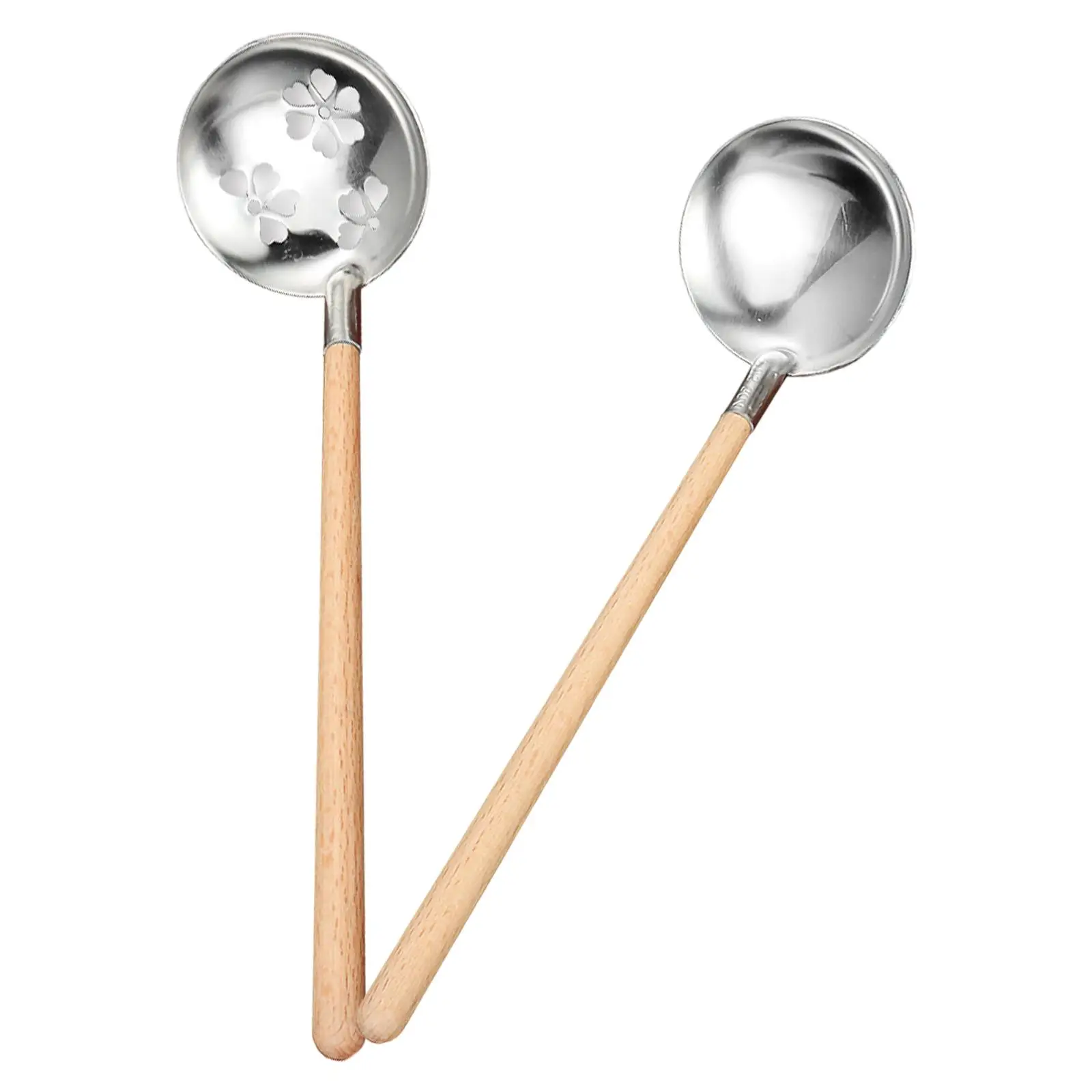This product photograph features two elegantly crafted utensils against a plain white background, each characterized by a light wooden handle and a round silver bowl at the end. The handle of the left utensil extends vertically upwards from the bottom of the image, culminating in a perfect, reflective silver circle adorned with an intricate floral design, featuring heart-shaped petals. The right utensil starts from the same point at the bottom of the photograph but diverges diagonally to the top right. Its handle, identical in size and color to the first, leads to a smooth, unembellished silver bowl. Both silver bowls catch and reflect the light, adding to the allure of these visually striking items. While their exact function remains ambiguous, their refined design and elaborate detailing suggest a blend of functionality and decorative appeal.